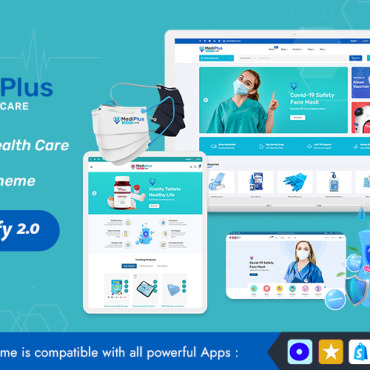This image appears to be a screenshot of a partially-visible webpage, possibly taken from a computer, phone, or tablet. The screenshot is cropped, cutting off some text and details around the edges. The main focus of the image is a medical-related content, featuring several elements:

1. **Central Main Content**:
   - There is a white container resembling a computer screen, showcasing a medical equipment website.
   - A woman is prominently displayed in green scrubs, wearing a blue and white face mask.
   - Adjacent to her image, there is a blue heart icon with the text "COVID-19 safety face mask."

2. **Product Listings at the Bottom**:
   - A list of purchasable items is shown:
     - The first item appears to be some type of medical chair.
     - The second item is blue, though its exact nature is unclear due to the cropping.
     - The next items listed are gloves and hand sanitizer.

3. **Secondary Image**:
   - Below the main content, there is another smaller box featuring a different woman in blue scrubs.
   - She is wearing a mask and a stethoscope around her neck, looking directly ahead.

4. **Left-hand Side Box**:
   - At the top of this box, there is an image of a bottle of pills, though the label is unreadable.
   - Below that, there are masks labeled "Med Plus":
     - Four white masks with blue handles.
     - One black mask with a light white handle.

Overall, the image conveys a medical-themed webpage focusing on COVID-19 safety products and features key visuals of healthcare professionals, safety masks, and other medical supplies.